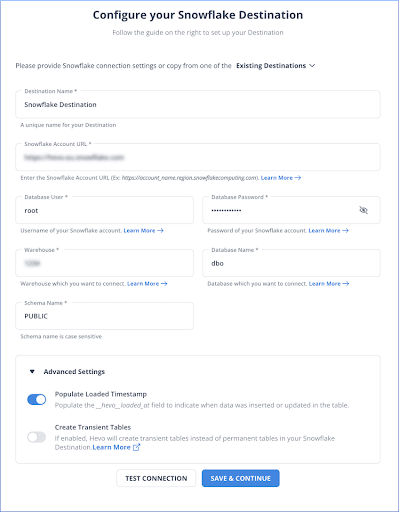The image depicts a webpage interface with a minimalist design, featuring a predominantly white background. At the top, centered in bold black text, it reads "Configure Your Snowflake Destination." Directly below this header, it instructs users to follow the guide on the right to set up their destination. The page then requests users to either provide Snowflake connection settings or copy from one of the existing destinations.

Highlighted in this section is a drop-down menu labeled "Existing Destinations." Below this, the interface prompts for a "Destination Name," accompanied by a text box where a unique name for the destination can be entered. Further down, another text box labeled "Snowflake Account URL," contains blurred-out text.

The form continues with several other text boxes for inputs such as "Database User," "Database Password," "Warehouse," "Database Name," and "Schema Name." Toward the bottom of the page, there is a drop-down menu labeled "Advanced Settings," which is indicated by a down arrow. Two advanced setting options are displayed: "Populate Loaded Timestamp" with a toggle switch in the 'on' position, illuminated in blue, and "Create Transient Tables."

At the very bottom of the interface, there are two central buttons. The button on the left, labeled "Test Connection," has black text on a white background, whereas the button on the right is blue with "Save and Continue" written in white text.